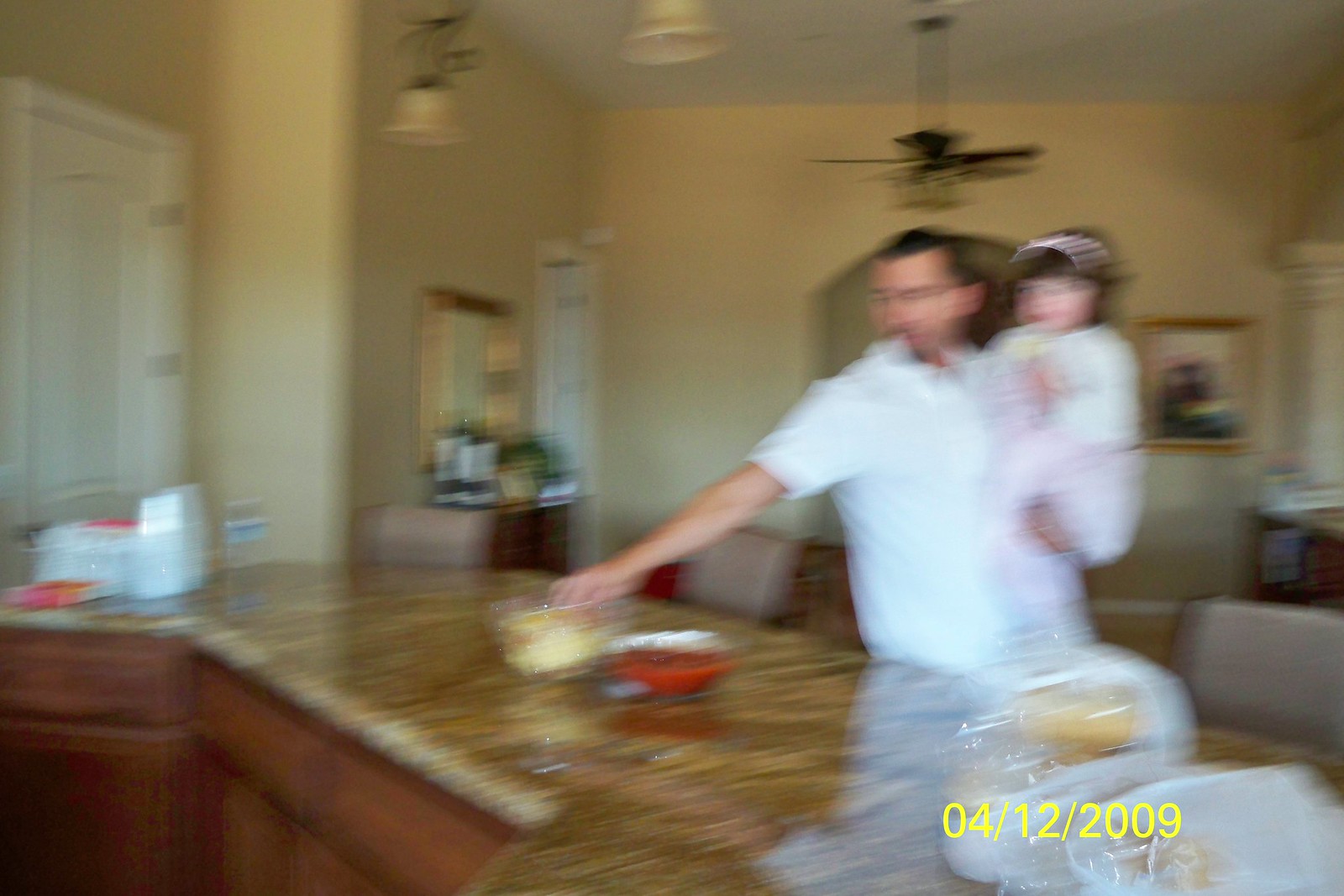The extremely blurry and out-of-focus photograph, dated 04-12-2009 in yellow text at the bottom right corner, depicts a room within a home featuring tan walls and a brownish-gold countertop. Beneath the countertop, there are dark brown wooden cabinets. In the background, a dark-colored ceiling fan is centrally located, with a painting situated just below it on the wall. To the right of the scene, a bookcase supports what appears to be a marble column. In the forefront, a man clad in a short-sleeved white shirt or chef's jacket is holding a child dressed in white pants, a white top, and a pink head covering. The man's right arm is extended towards a bowl on the countertop, possibly reaching for popcorn or chips.